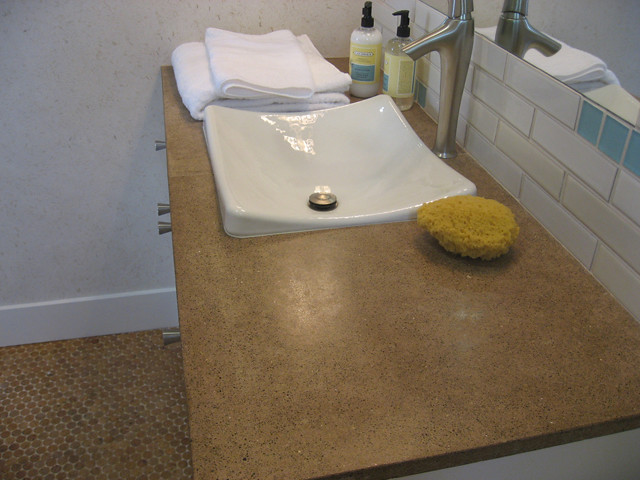This photo showcases a meticulously designed bathroom vanity area. The floor is adorned with small, circular brown tiles, adding a touch of texture and warmth to the space. The walls are painted white and accented with white baseboards for a clean look. The vanity features a medium brown countertop that stretches across the width of the photo, providing ample surface area. 

At the center of the countertop sits an elegant sink with a gold round stopper at its base. The sink basin subtly dips in the middle and ascends gracefully towards the edges. Adjacent to the sink, a teardrop-shaped natural yellow sponge rests on one side, while on the other side lies a neatly folded white hand towel. Behind the towel, two clear pump bottles with black pumps and yellow labels sit side by side, likely containing soap and lotion. 

A tall, stainless steel faucet is mounted behind the sink, providing a modern, sleek touch. The backdrop of this vanity includes a white ceramic tile wall, extending up to a large mirror that spans the entire length of the countertop, contributing to the room's airy and spacious feel. The mirror reflects the bathroom's carefully coordinated elements, enhancing the overall aesthetic appeal.